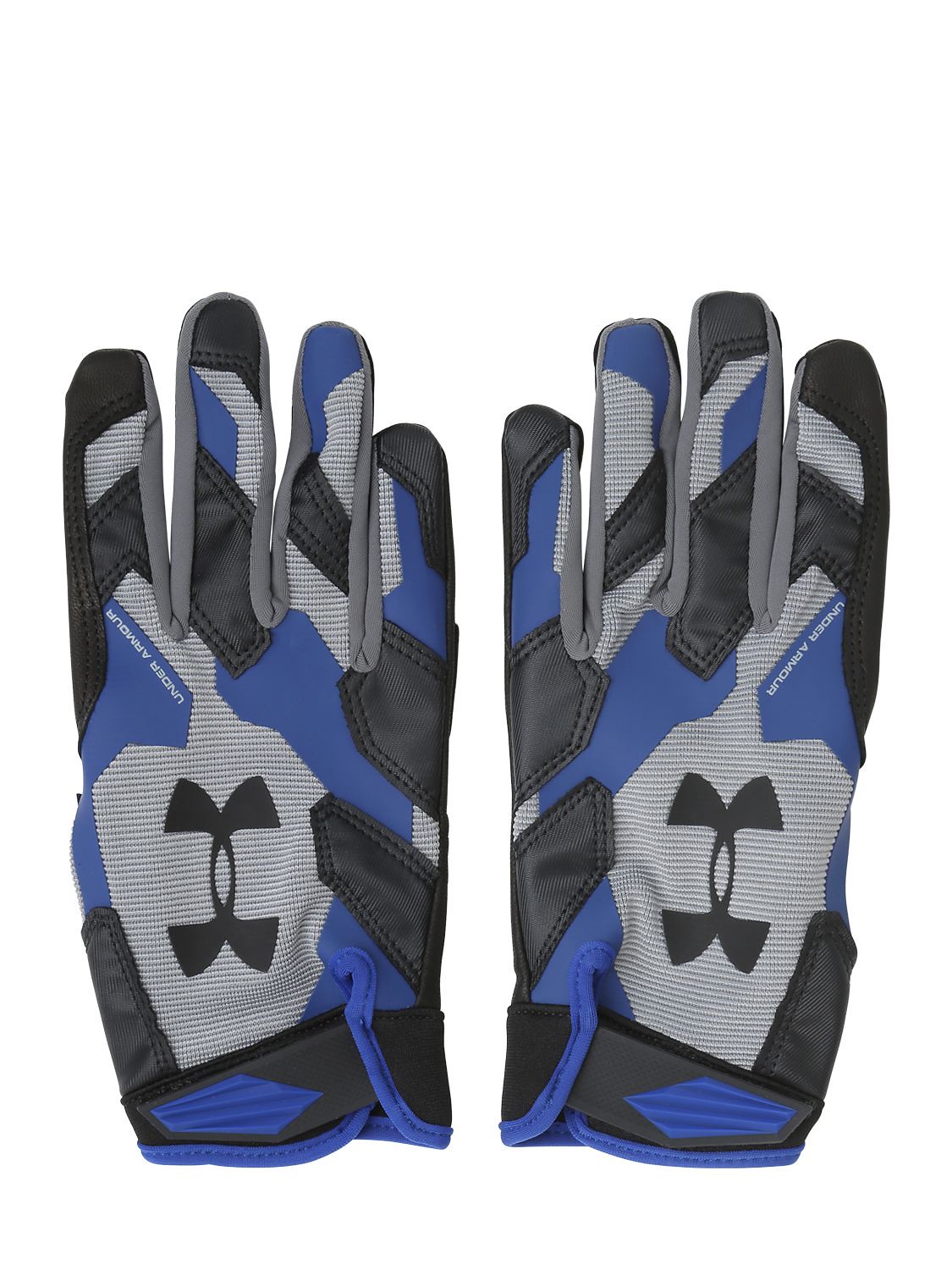This image features a pair of Under Armour gloves set against a completely white background. The gloves are positioned palm down, with the left glove on the right side of the image and the right glove on the left. This reversal creates a mirrored effect. Both gloves are primarily designed with a pattern of black, grey, and blue. The gloves feature grey mesh backing with black leather patches and medium blue fabric pieces scattered across the surface. The Under Armour logo is prominently displayed on the grey area at the back of each hand, oriented vertically. The index, middle, and pinky fingers have black leather tips, while the ring finger has a blue and grey covering. The thumb portions of the gloves are not visible as they are tucked underneath. At the base of the gloves, there is a black Velcro strap with blue patches, ensuring an adjustable fit. The gloves could be suitable for sports, work, or promotional use, but the specific type is not defined.